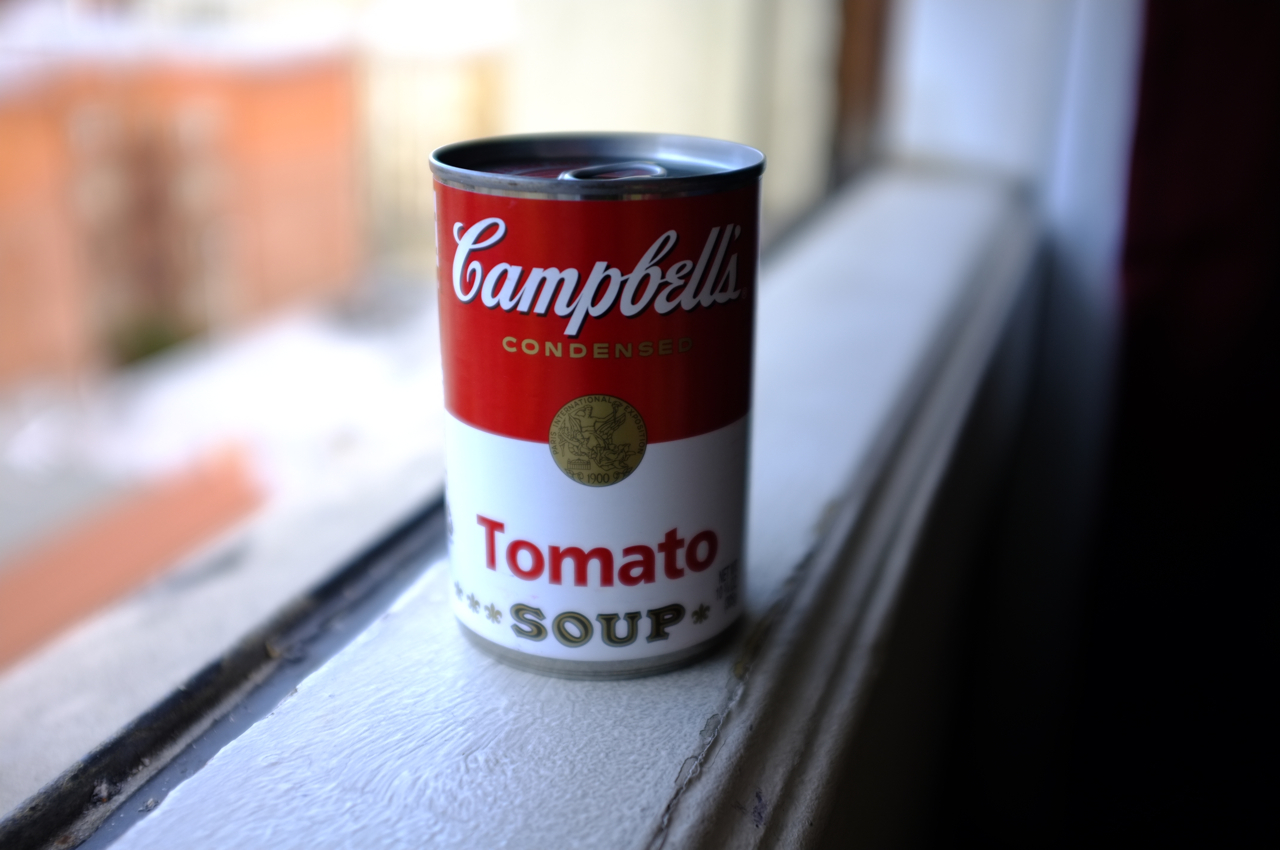In this visually striking image, we see a classic can of Campbell's condensed tomato soup prominently positioned on a pristine white ledge beside a window. The iconic Campbell's branding is showcased with 'Campbell's' elegantly written in white cursive letters at the top of the red and white label. Below this, the word 'condensed' is printed in small gold letters. Central to the design, a gold medal emblem adorns the middle of the can, adding a touch of historical distinction. The word 'tomato' appears in bold red letters, followed by the word 'soup' in a softer gold hue beneath it. The can's metallic top, featuring a convenient pull-tab mechanism for easy opening, glints subtly in the light. On the left side of the image, the background blurs into the scene outside the window, where a vague outline of a building is discernible, further emphasizing the focus on the iconic can of soup.